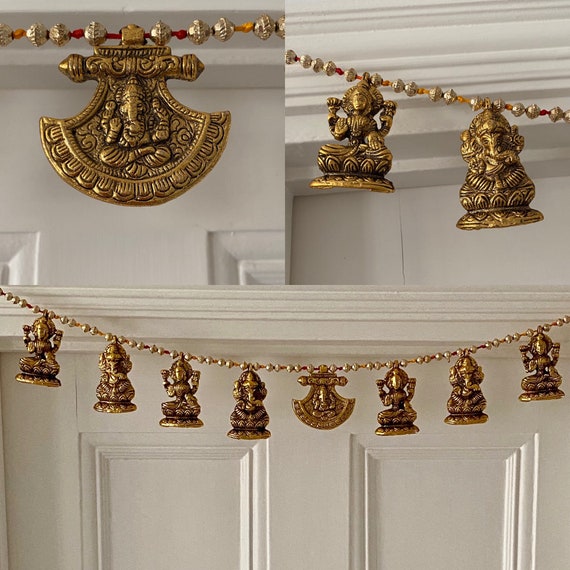The image depicts an elaborate, ornate string draped across a white paneled door. The string, reminiscent of a decorative necklace, is crafted from interconnected metal balls, from which hang various intricately detailed bronze charms. Central to the string is a larger medallion, possibly gold-toned but more likely bronze, featuring a shield-like design with a slightly unsettling figure. Flanking this centerpiece are numerous miniature statues, some resembling Buddhas or ancient oriental figures, with four visible on the left and three on the right, though the string may extend beyond the photographed portions. The fine detailing of each figure is accentuated by black highlights in the crevices. The string also appears to incorporate small yellow and red beads, adding to its ornate complexity.